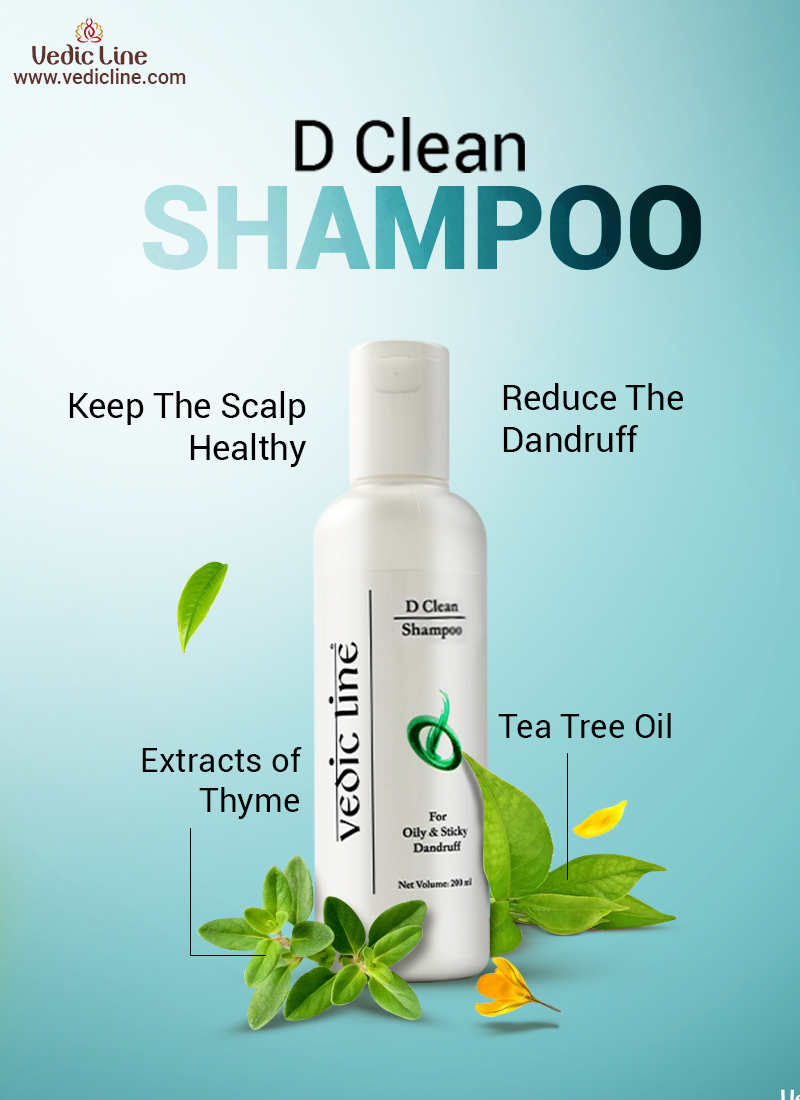This advertisement for DeClean Shampoo by VedicLine features a prominent display of a white shampoo bottle adorned with the VedicLine logo, aligning vertically. The composition is accentuated with detailed text in black and bluish font, prominently showcasing "DeClean Shampoo" at the center. This shampoo is specially formulated for oily and sticky dandruff and aims to keep the scalp healthy while reducing dandruff. The top-left corner highlights the VedicLine logo and their web address, www.vedicline.com. Surrounding the base of the bottle are leafy illustrations, designated with arrows; one points to "extracts of thyme" and the other to "tea tree oil," indicating the natural ingredients used in the formulation. The bottle itself features a sleek design in blue and white, with green accents depicting the tea tree leaves. The ad's clear emphasis on natural extracts suggests a focus on effective dandruff reduction using herbal ingredients.